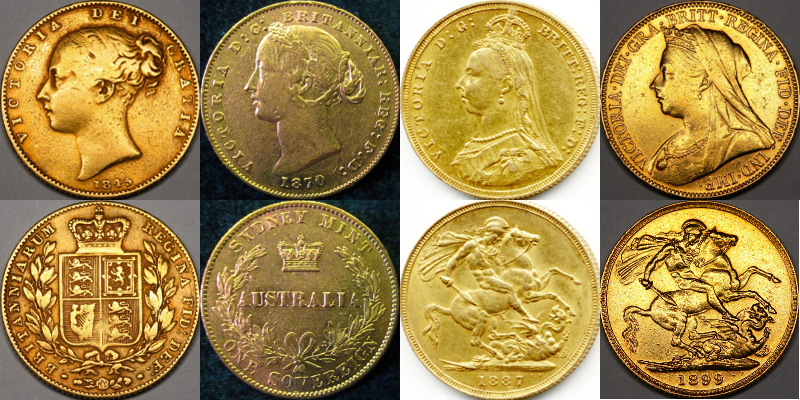The image is a horizontally aligned rectangular display featuring the front and back sides of four different gold coins. Each coin occupies a distinct slot in this arrangement: the top row showcases the obverse (front) sides and the bottom row displays the reverse (back) sides.

The coins on the far left are set against a dark gray background on top and a lighter gray background on the bottom. This coin, dated 1846, has "Victoria D-E-I-C-R-A-T-I-A" inscribed along the edge, with the profile of Queen Victoria facing left. The reverse features a shield crowned with a smaller inscription surrounding it.

The second coin from the left is on a black background on top and a medium gray background on the bottom and is marked 1870. It shows another depiction of Queen Victoria with "Victoria D-G-B-R-I-T-T-A-N-R-R-V-T-R" prominently visible. The reverse side bears the inscription "Australia" and "Sydney Mint" at the top, "One Sovereign" at the bottom, and also features a wreath.

The third coin is on an off-white background on top and a white background on the bottom. While the date is obscured, it features the profile of Queen Victoria at a later stage, signified by additional regalia. The reverse has an image of a horseman with a sword, dated either 1837 or 1887.

The last set of coins, situated on a dark gray background on top and a lighter gray background on the bottom, is dated 1899. The obverse displays Queen Victoria adorned with elaborate jewelry including a full crown, headdress, and earrings. The reverse side continues the motif of a horseman with a sword, similar to the earlier coin.

These coins, varying in age and design details, reflect different stages of Queen Victoria's reign and are unified by their gold composition.